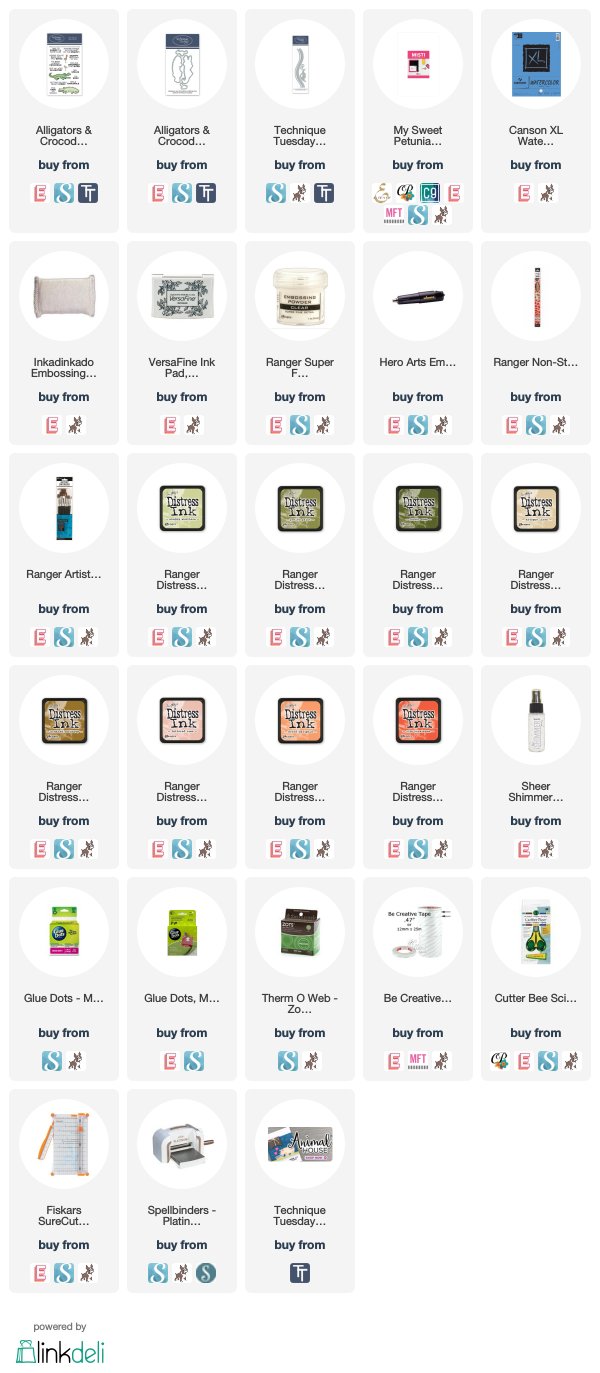The image displays a search result captured on a mobile phone, showcasing a variety of craft supplies available for purchase online. The list includes:

1. **Alligators and Crocodiles** - A potential name of a game or product, with another listing for the same item available from the same vendor.

2. **Technique Tuesday** - Listed below the previous item.

3. **My Saved Petunia** - Appears to be another crafting product.

4. **Carson XL Water** - Partially visible, the full name is unclear.

5. **Inkadinkado Embossing** - Likely a type of embossing tool or material.

6. **VersaFine Ink Pad** - Various inks for stamping.

7. **Ranger Super** and **Hero Arts Film** - Crafting supplies, potentially inks, films, or similar materials.

8. A series of **Ranger products** including **Ranger Distress** items, shown multiple times with variations in colors. 

9. **Shiner Shimmer** - Another crafting item that adds shine or shimmer to projects.

All products appear to be presented by **Link Deli**, an online platform from which these items can be purchased.